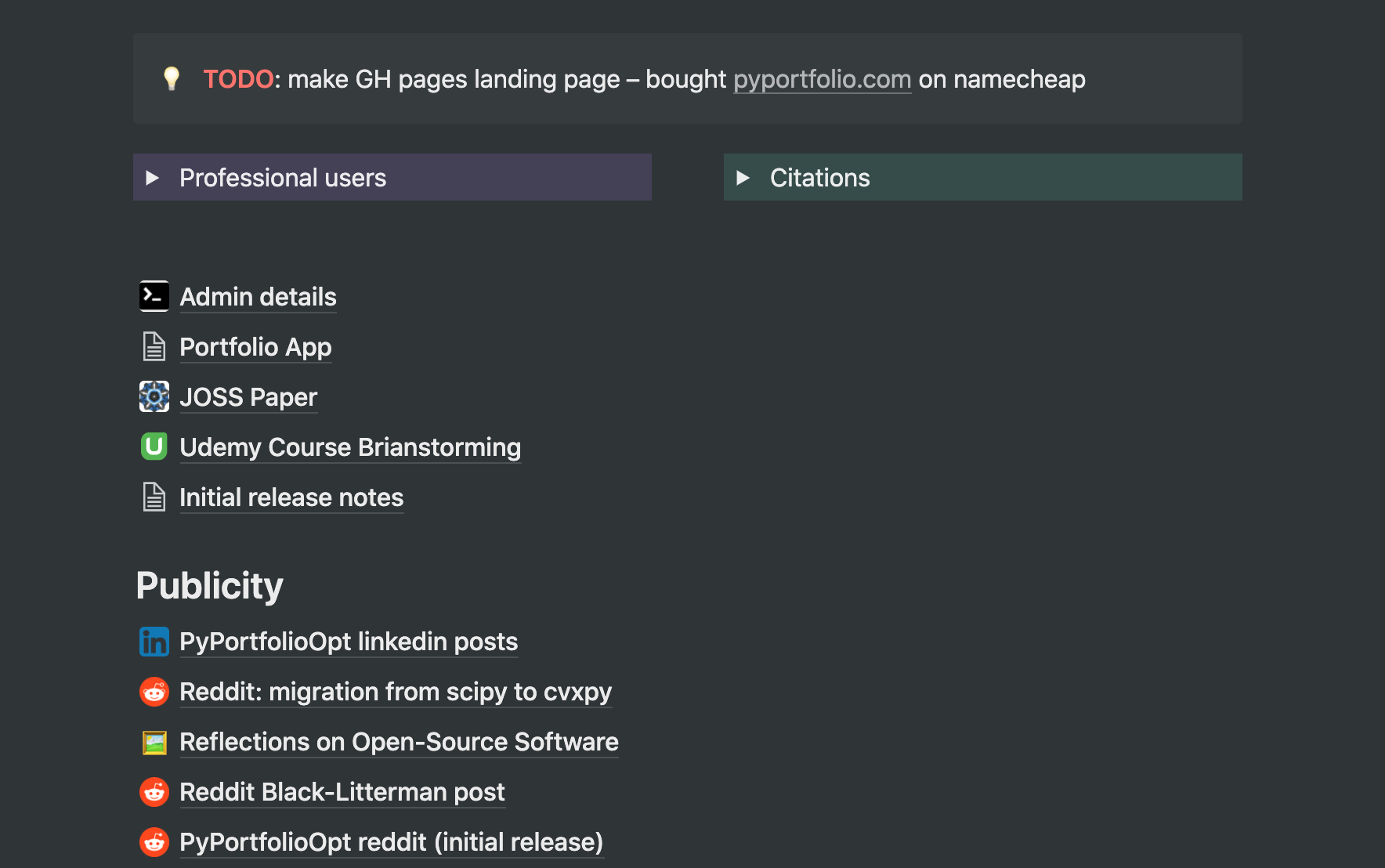Here's a cleaned-up and detailed caption for the image:

---

The image features a promotional landing page designed against a sleek black background. The title "HighPortfolio.com" is prominently displayed in gray on a name sheet. Key sections are color-coded for clarity: "Professional Users" is highlighted in white on a purple rectangle, "Citations" in white on a green medium-gray rectangle, and "Admin Details" in white. Notable content includes "Portfolio App," "JOSS Paper," "Udemy Course Brainstorming," "Initial Release Notes," and "Publicity." The branding "HighPortfolioOpt" is uniformly stylized with both 'P's and the 'O' capitalized. The image also references strategies and milestones like LinkedIn posts, Reddit activities, migration from Spicy to CVXPY, reflections on open-source software, and other key items such as "Reddit Black-Dash," "Litterman Post," and initial release notes for "PopPortfolioOp" (with both 'P's and 'O' capitalized).

---